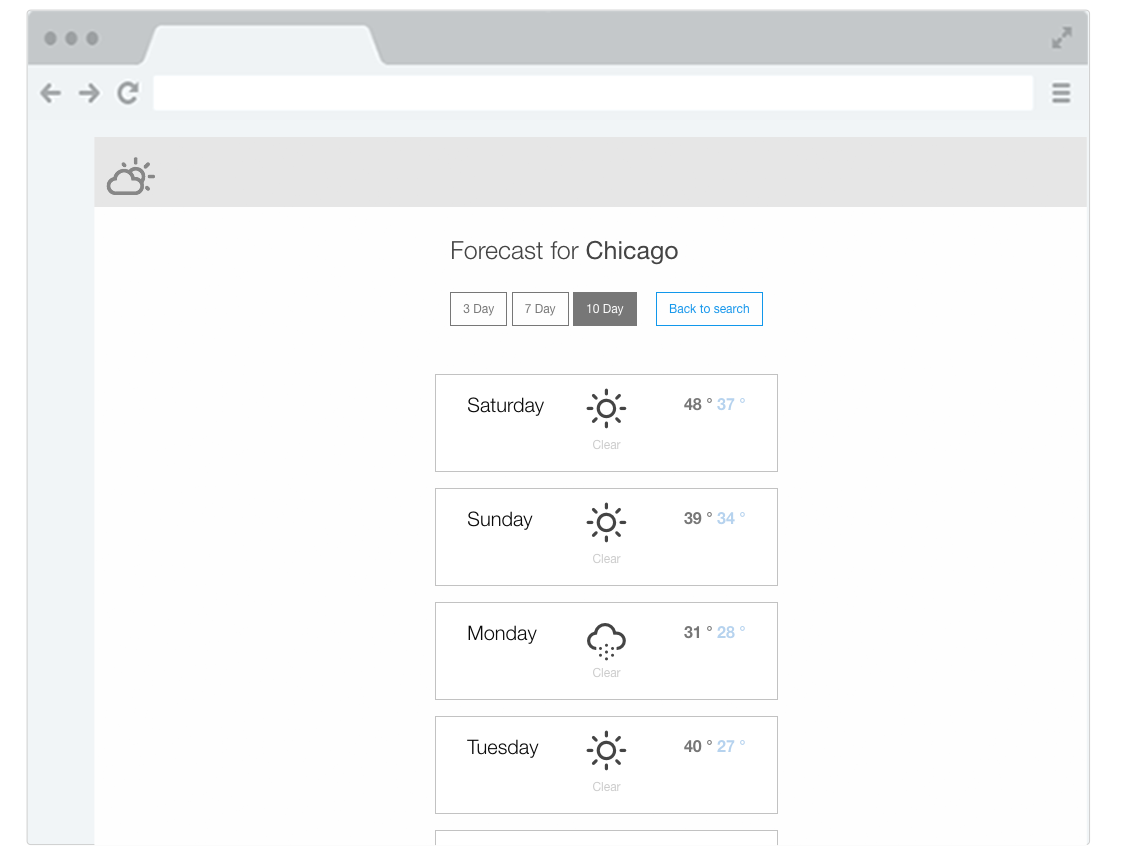This image is a screenshot of a web browser tab on a computer. At the top, there is a light gray toolbar area, featuring three darker gray circles on the left. The browser window contains a search bar, which is also light gray, positioned beneath the toolbar. On the left side of the search bar, there are navigation buttons: a left arrow, a right arrow, and a refresh icon. To the right of the search bar, three horizontal lines are displayed, likely representing a menu or options button.

Directly below the search bar is a white box displaying the text "Forecast for Chicago." Underneath this box are four selectable options labeled: "3 Day," "7 Day," "10 Day," and "Back to Search." Below these options, detailed weather information for the upcoming days is provided.

For Saturday, the weather forecast shows clear skies with sunshine. On Sunday, it remains clear and sunny with a temperature of 39 degrees. Monday’s forecast depicts clear skies with some clouds, accompanied by a temperature of 31 degrees. Finally, Tuesday's forecast returns to clear, sunny conditions with a temperature of 40 degrees.